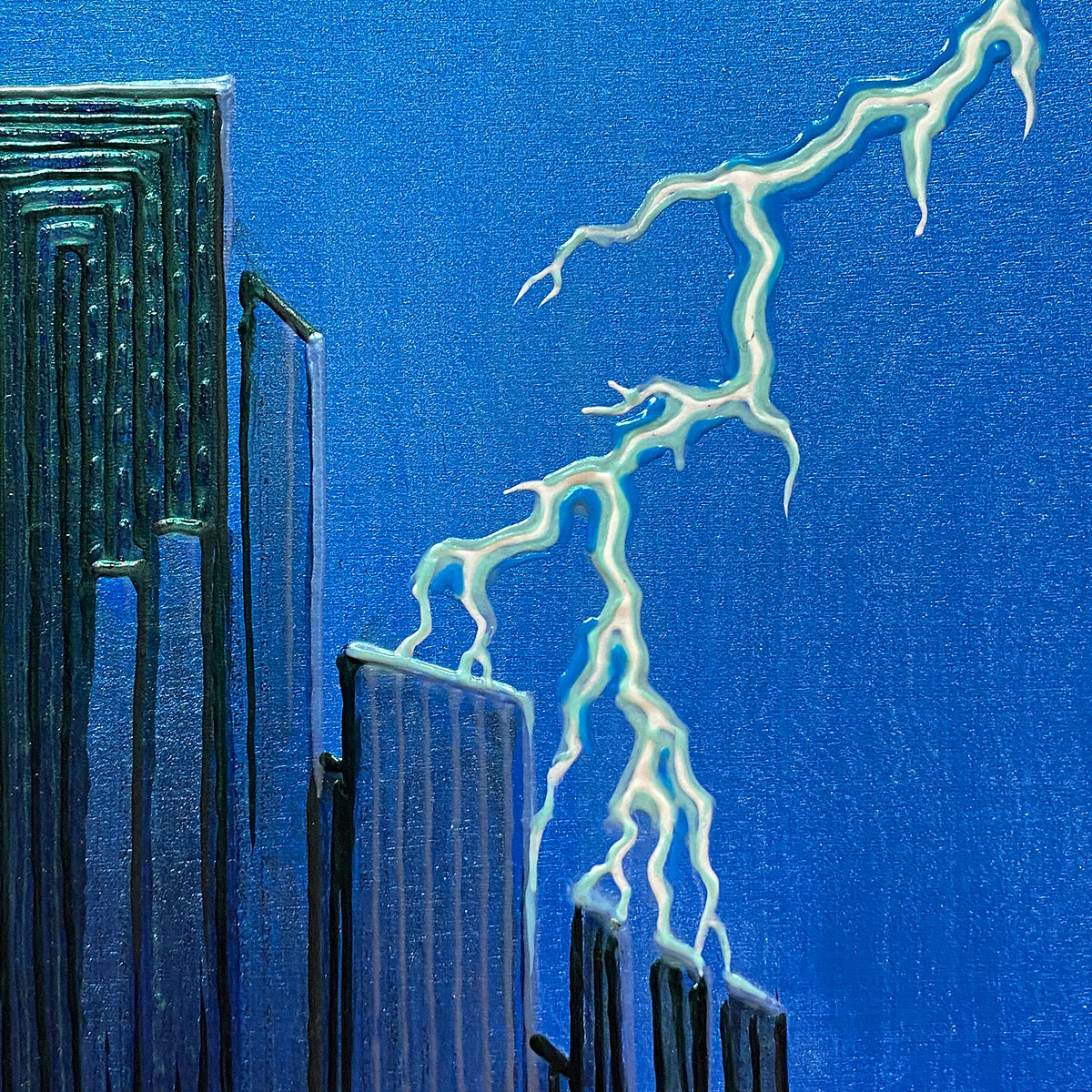This detailed painting depicts a dramatic scene of lightning striking a cityscape, characterized by bold, textured brushstrokes, suggesting it is an oil painting. The background is a vivid, bright blue, representing the sky, with a textured pattern that evokes a sparkling effect. From the upper right corner, a stark white lightning bolt, edged with light blue, descends and makes contact with the tops of several buildings, including one with distinctive vertical grey lines and another smaller trio of navy structures below.

On the left side of the painting, a high-rise building stands dominant, rendered in dark navy blue with layers of dark green, transitioning to shorter buildings with slanted rooftops painted in a metallic green hue. Some of these structures also display silver lines, possibly mimicking the look of windows. The tallest building, rectangular in shape, is bordered in different shades, creating a layered visual effect, while below it, other buildings are illustrated in royal blue with silver accents.

The overall cityscape presents a mix of architectural forms, blending tall and shorter buildings with varied textures and colors, seamlessly integrated into the scene. The right side of the painting remains primarily the bright blue sky, contrasting starkly with the electrifying strike of the lightning and the dark, metallic tones of the city below.